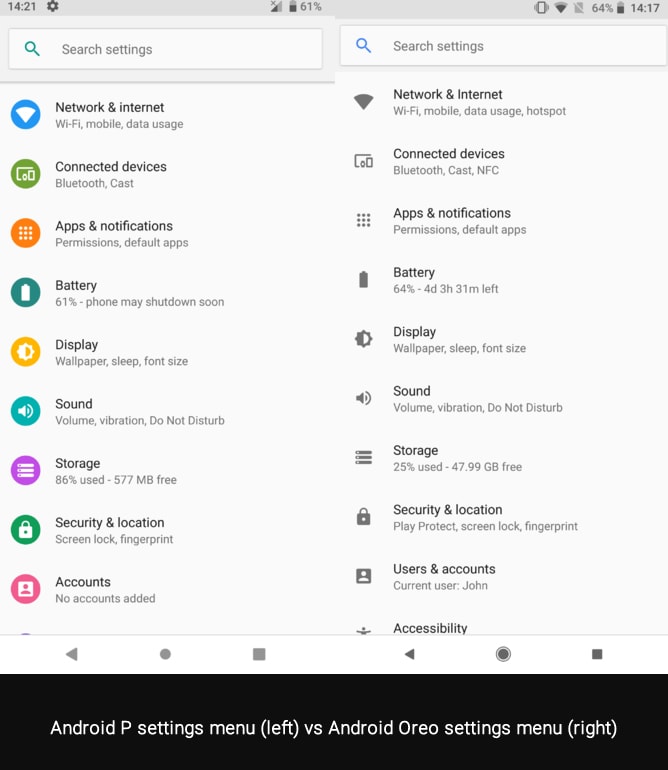Screenshot comparison of Android P vs. Android Oreo settings menus. The left side of the image showcases the settings menu from Android P, characterized by vibrant, colorful icons within circular backgrounds. For example, the "Network and Internet" option features a blue circle with a white cheese wedge icon, and the "Connected Devices" option displays a green circle with a white outline of a connected device. In contrast, the right side of the image presents the settings menu from Android Oreo, where all icons appear in grey scale without any colorful backgrounds. This comparative screenshot highlights the design evolution between Android P and Android Oreo, emphasizing the shift from a colorful interface to a more monochromatic and minimalist design approach.